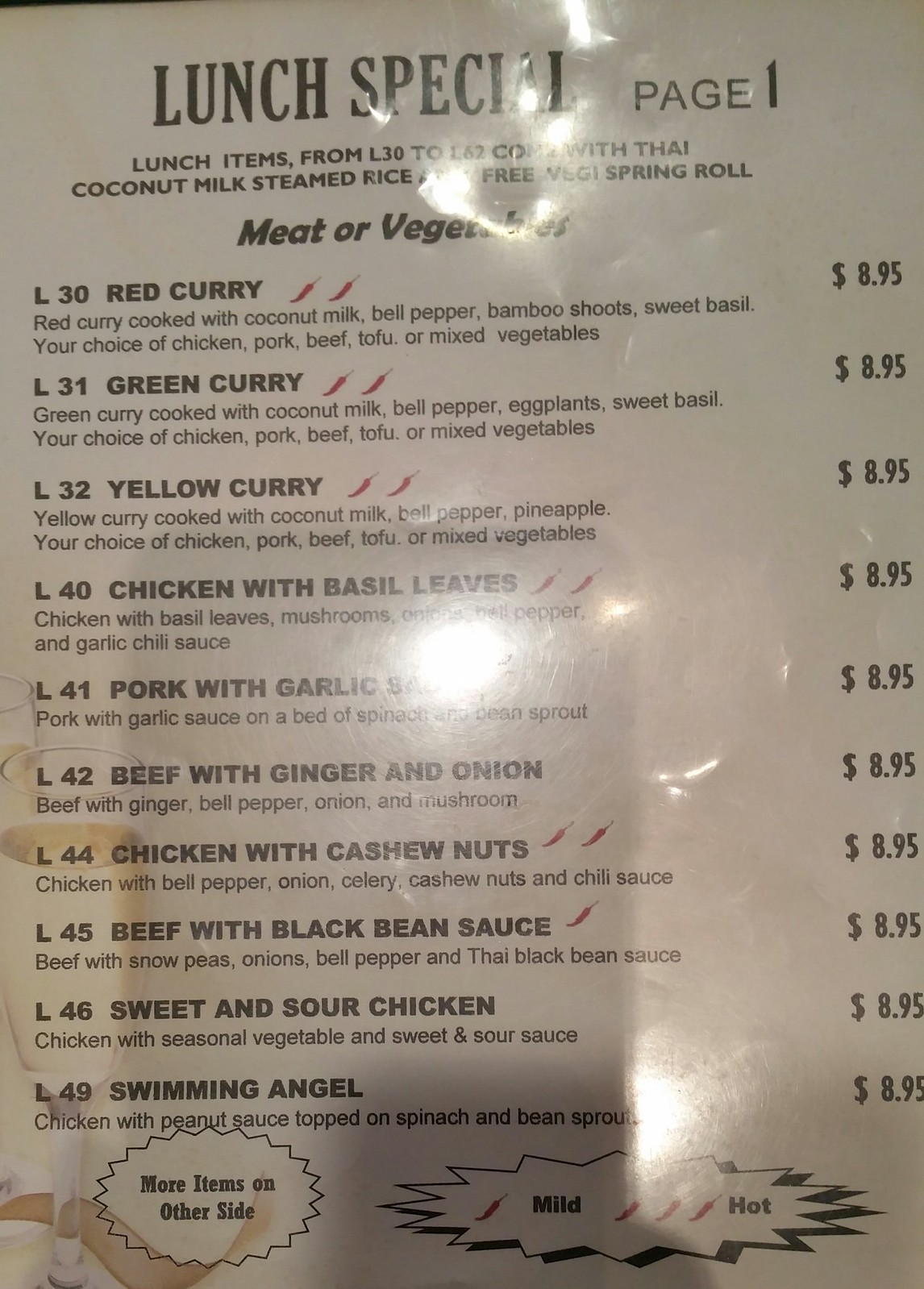The image features a detailed close-up of a lunch menu at a restaurant. The menu's layout is set against a white background with black text. At the top, it prominently reads "Lunch Special" and "Page 1," indicating the current section of the menu. 

The menu offers lunch items numbered from L30 to L62, each of which is paired with Thai coconut milk, steamed rice, and a complimentary veggie spring roll.

Here are the featured dishes with descriptions and prices:

- **L30: Red Curry**: A savory dish cooked with coconut milk, bell pepper, bamboo shoots, sweet basil, and your choice of chicken, pork, beef, tofu, or mixed vegetables. Price: $8.95.

- **L31: Green Curry**: A flavorful option prepared with coconut milk, bell pepper, eggplants, sweet basil, and your choice of chicken, pork, beef, tofu, or mixed vegetables. Price: $8.95.

- **L32: Yellow Curry**: This dish includes coconut milk, bell pepper, and pineapple, with options of chicken, pork, beef, tofu, or mixed vegetables. Price: $8.95.

Additionally, various non-curry dishes are listed, each priced at $8.95:

- **L40: Chicken with Basil Leaves**: Sautéed chicken with basil leaves, mushrooms, bell pepper, and garlic chili sauce.

- **Pork with Garlic**: Pork served on a bed of spinach with bean sprouts, topped with garlic sauce.

- **Beef with Ginger and Onion**: A combination of beef, bell pepper, onion, and mushroom enhanced with ginger.

- **Chicken with Cashew Nuts**: Chicken mixed with bell pepper, onion, celery, cashew nuts, and chili sauce.

- **Beef with Black Bean Sauce**: Beef paired with snow peas, onions, bell pepper, and Thai black bean sauce.

- **Sweet and Sour Chicken**: Chicken cooked with seasoned vegetables in sweet and sour sauce.

- **Swimming Angels**: Chicken served with peanut sauce over spinach and bean sprouts.

Each dish reflects the rich, bold flavors characteristic of Thai cuisine and offers a variety of protein and vegetable options to cater to different preferences.